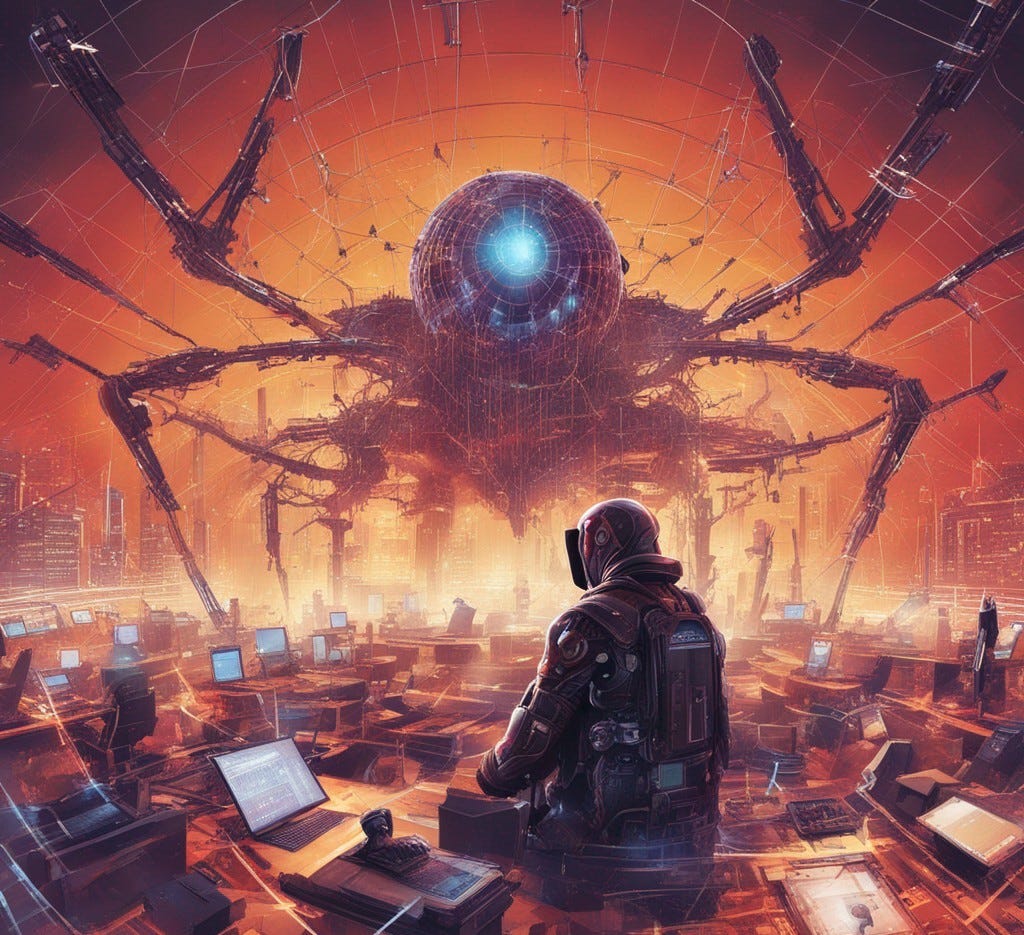This is a highly detailed, computer-generated, color sci-fi illustration set within a large, domed structure. In the top two-thirds of the square image dominates a giant mechanical spider, which is facing the viewer. The spider has a rounded, globe-shaped head with a bright blue light at the top, enhancing its formidable and high-tech appearance. Its multiple appendages, with bendable joints, extend both upward and downward, making it look as though it is stomping throughout the environment. The building's domed roof presents a gradient of dark orange to light orange hues, adding a dramatic backdrop.

Surrounding the spider are numerous computer setups with lit monitors scattered throughout the room, though the details on the screens remain indistinguishable. Flanking the composition, slightly out of focus, is the silhouette of a city skyline visible on either side of the image, enhancing the scene's futuristic ambiance.

In the foreground, slightly off-center to the left, is a lone individual. Clad in black and gray protective outerwear complete with a face mask and visor, the figure's back is turned towards the viewer. The individual's ambiguous posture, obscured by a hazy and blurry atmosphere near the bottom of the image, leaves it uncertain whether they are standing or sitting. The protective suit features a flat, backpack-like extension, adding to the sci-fi narrative of the illustration.